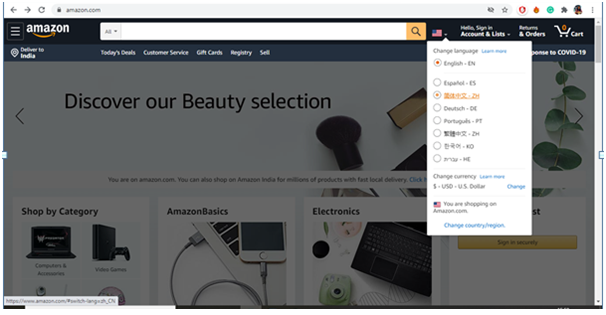The image depicts an Amazon website interface with a darkened background, created by an active pop-up window. At the top of the page, there is a navigational toolbar featuring a left arrow key, a right arrow key, and a refresh button, all set against a white background. The address bar in the toolbar displays "amazon.com," followed by a star icon, an information symbol (denoted by an 'i'), and additional icons.

Just below the address bar, the Amazon logo is visible alongside a drop-down menu for various settings. The menu includes a search bar and an American flag icon, signifying the current language preference. When expanded, the drop-down menu reveals language options such as English (EN), Español (ES), Dutch (DE), and Portuguese. Additionally, there are several options marked by non-Latin script symbols.

Further down, the pop-up window offers currency options under the "Change currency" section. It currently displays the US dollar (USD) as the selected currency, with an option to change it. Below this, the pop-up confirms that the user is shopping on amazon.com and provides a link to change the country or region, highlighted in blue text.

Overall, the image captures the intricacies of user navigation and customization settings available on the Amazon website interface.